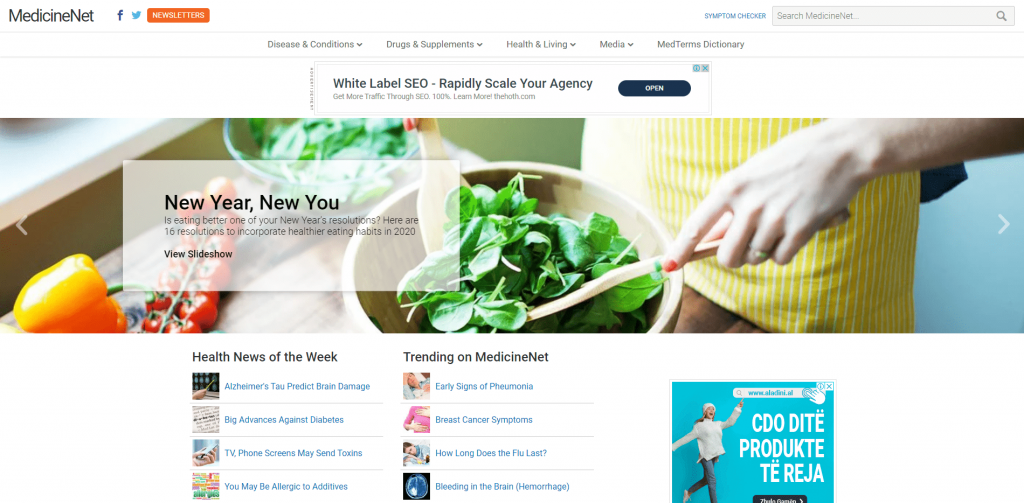This is a detailed caption of an image from the MedicineNet website:

---

The MedicineNet website homepage features a prominent advertisement for "White Label SEO" services with the tagline "Rapid Scale Your Agency." The site includes various drop-down menus, though the text is notably small and somewhat difficult to read. At the center of the page, a large banner image showcases a woman preparing a spinach salad, accompanied by the text "New Year, New You" and a prompt to "View Slideshow." This suggests a collection of recipes and healthy eating tips targeted at new year's resolutions. The bottom section of the page highlights links to the "Health News of the Week" and "Trending on MedicineNet," indicating regularly updated content on health and wellness. Additionally, another advertisement in a foreign language, reading "CDO Diet Produktivitiera," is located in the lower right corner of the page. Overall, the website is a resource focused on promoting healthier lifestyles through informative articles and practical advice.